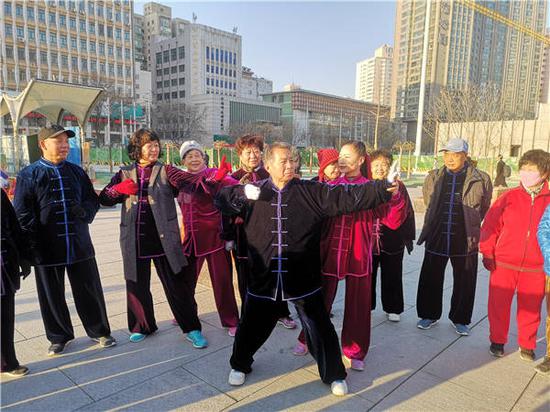In a bustling downtown area, possibly Hong Kong or another city in Asia, a striking scene unfolds as a group of Chinese people gather in a circle. At the center stands a middle-aged man with a black Chinese outfit adorned with a purple accent trim, including six horizontal purple lines down the front of his shirt. His pose suggests he is practicing Tai Chi, drawing an imaginary bow in the air with his left arm extended and right arm bent. Around him, the group, consisting of men and women of various ages, some emulating his pose, are dressed in similarly styled attire. The colors vary with individuals in black, purplish-pink, and red gis, including a lady in a red jacket and pants with short hair, and an older gentleman wearing a blue hat. The surroundings, marked by tall, multi-story buildings, add a sense of urban vibrancy to the photograph, as the participants seem to engage in a harmonious practice session beneath the towering cityscape.